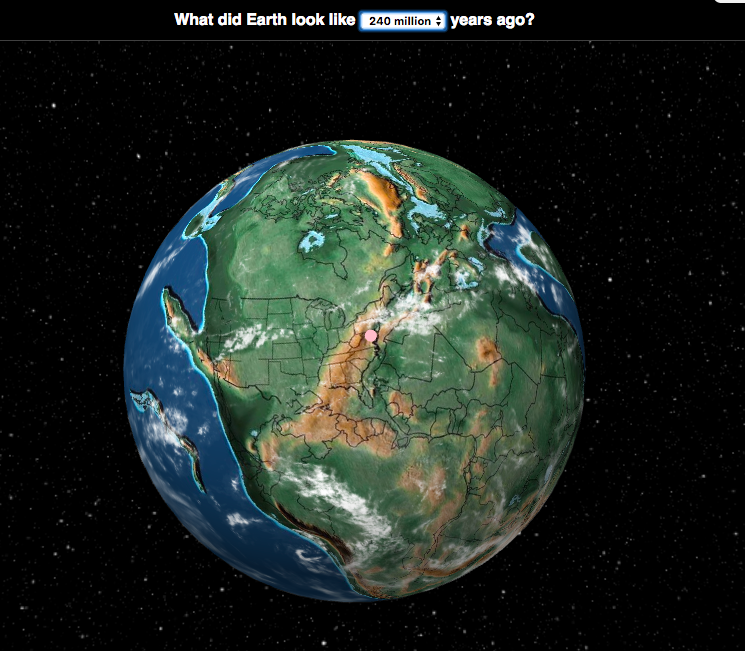The image features a CGI representation of Earth set against a black background speckled with tiny white dots, mimicking the vastness of space. At the top of the image, a caption reads, "What did Earth look like 240 million years ago," accompanied by a radio button with arrows, suggesting the ability to scroll through different time periods. Dominating the center of the image is a large depiction of the globe, showcasing an extensive green landmass reminiscent of the supercontinent Pangea. This landmass prominently displays the geographical outlines of current countries such as the United States, Canada, and Mexico, indicating their historical positions. Surrounding this primary landmass are diverse regions including mountainous areas and deserts, and small islands scattered across the adjacent oceans. There's also minimal cloud cover visible. Additionally, a light pink dot is marked near the middle of the landmass, though its significance is unclear. The overall visual effectively illustrates the Earth's prehistoric configuration, with the continents connected in a way that contrasts sharply with their present-day separation.